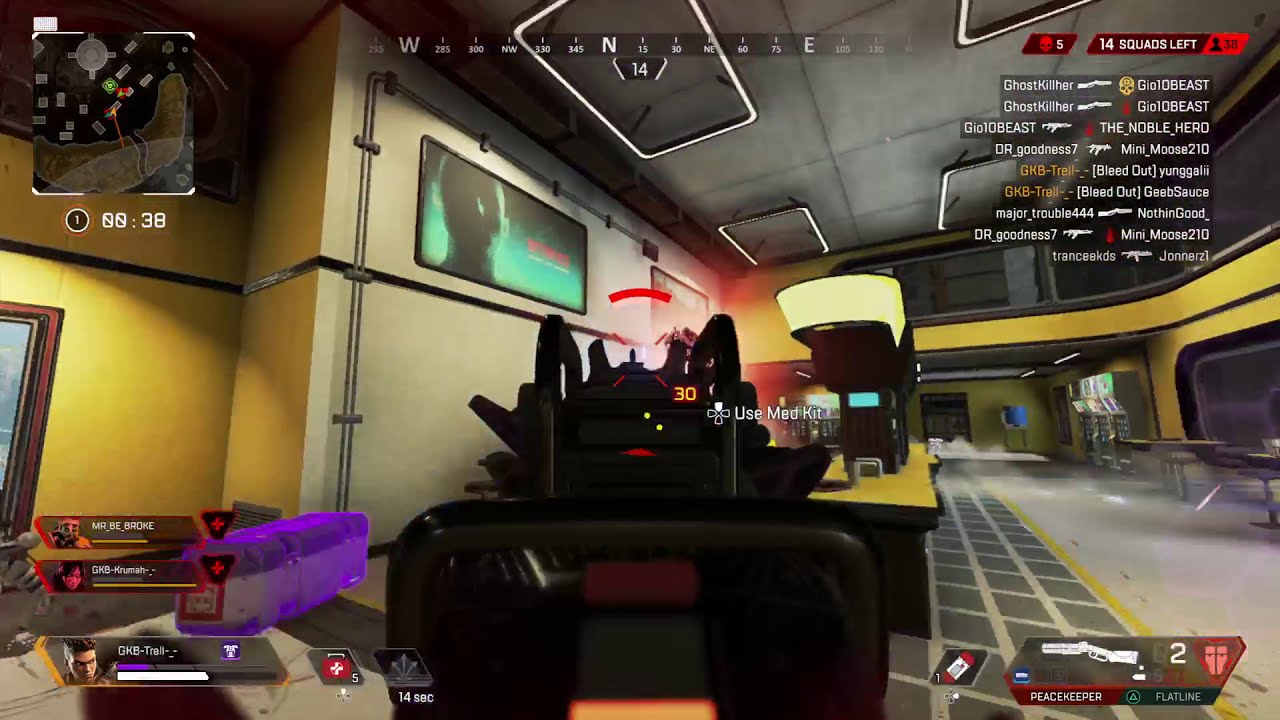This horizontally aligned rectangular image is a still shot from a video game scene taking place inside an alien-looking building. The right side of the building features white tile, transitioning to a checked gray-and-white tile pattern in the middle to the left side. A yellow wall is visible on the far left, and the ceiling consists of large square gray tiles. Centrally, there's a table with a yellow top, holding various unspecified items. Dominating the foreground is a black vehicle, resembling a four-wheeler, with the text "Use Med Kit" near it. 

In the lower left corner, there are icons displaying three character images accompanied by unreadable white text naming the characters. The upper right corner of the image indicates "14 squads left" with a skull icon followed by the number five, alongside several player names and their tags, including Ghost Killer, Geo Ten Beast, Oh Our Goodness, and GK Betrayal. Additionally, there are rifle icons, possibly suggesting weapon allocations or kills. The lower right corner shows a gun labeled Peacekeeper, with two of such guns present.

A square overview map is located in the upper left corner, and a compass is centered at the top of the screen. The scene suggests that the characters are engaged in an intense multiplayer battle, possibly in the process of healing, as indicated by the "Use Med Kit" prompt.